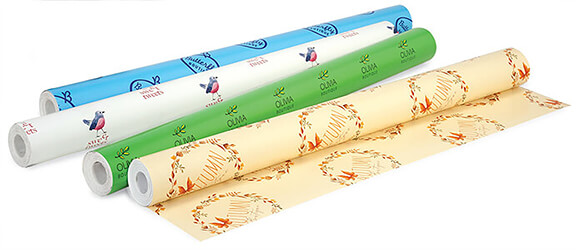This photograph captures four distinct rolls of gift wrapping paper, each with unique designs, set against a plain white background, reminiscent of a product image from an online shopping catalog. The roll in the foreground features a cream-colored design adorned with wreaths of leaves and the word "autumn" prominently displayed, giving it an elegant fall theme. Next, there is a vibrant green roll decorated with a repeated pattern of yellow leaves and the name "Olivia," suggesting a custom design. The third roll is white and features a charming pattern of bluebirds interspersed with unreadable text, adding a playful touch. The final roll in the set is a baby blue paper, simple yet classic. Each roll appears to be about an inch and a half thick, showcasing the intricate and varied designs, perfect for a range of gift-giving occasions.